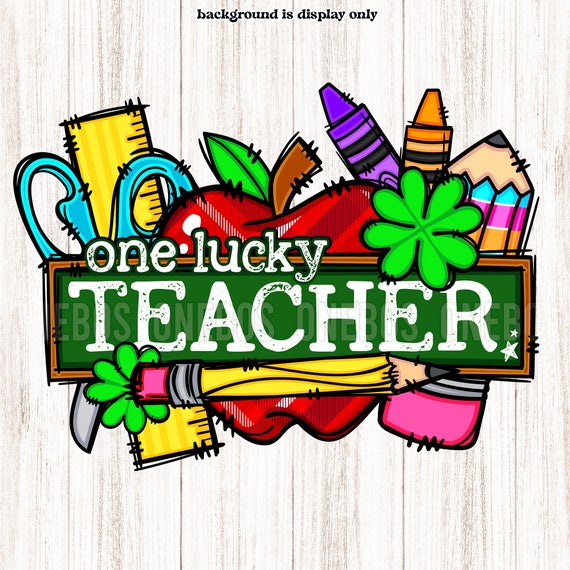The image appears to be a vibrant advertisement or digital logo with a St. Patrick's Day theme set against an artificial vertical wood grain background in off-white with slight brown texture. At the very top, there's a small inscription stating "background is display only." The center of the image is adorned with various colorful school supplies including blue scissors, a yellow ruler, a large red apple, purple and orange crayons, a colorful pencil, and a standard yellow pencil with a pink eraser. Amidst these items, there are two four-leaf clovers symbolizing luck. Over the collage of items, the text "one lucky teacher" is prominently displayed. The words “one lucky” appear in white letters above a green rectangle framed in brown, resembling a chalkboard, which carries the word “teacher” in large white letters. Overall, the composition is highly stylized, giving off a playful, clip-art aesthetic.